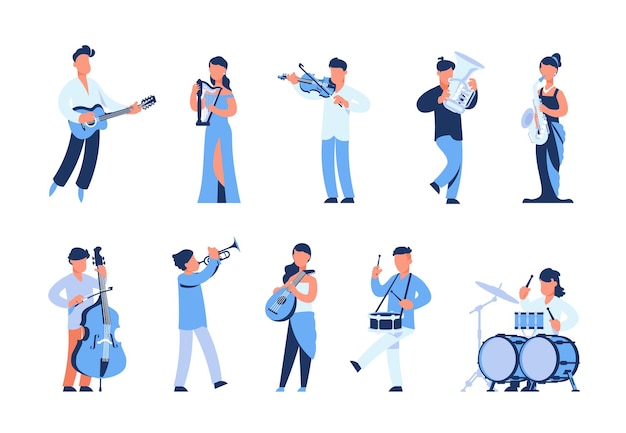The image features a white background with a detailed illustration of 10 different faceless, cartoon-like people, each depicted in shades of blue and light blue, against a backdrop devoid of any text or other elements. The people are all playing various musical instruments and have a uniform tan salmon color. In the top row, from left to right, there is a man playing a guitar, a woman playing a harp, a person playing a violin, a person playing a tuba, and a woman playing a saxophone. In the bottom row, a man is playing a cello, a woman is playing a trumpet, another woman is strumming a ukulele, a man is playing a drum, and a woman is seated at a larger drum kit. All figures and their instruments are rendered in the same blue color palette.